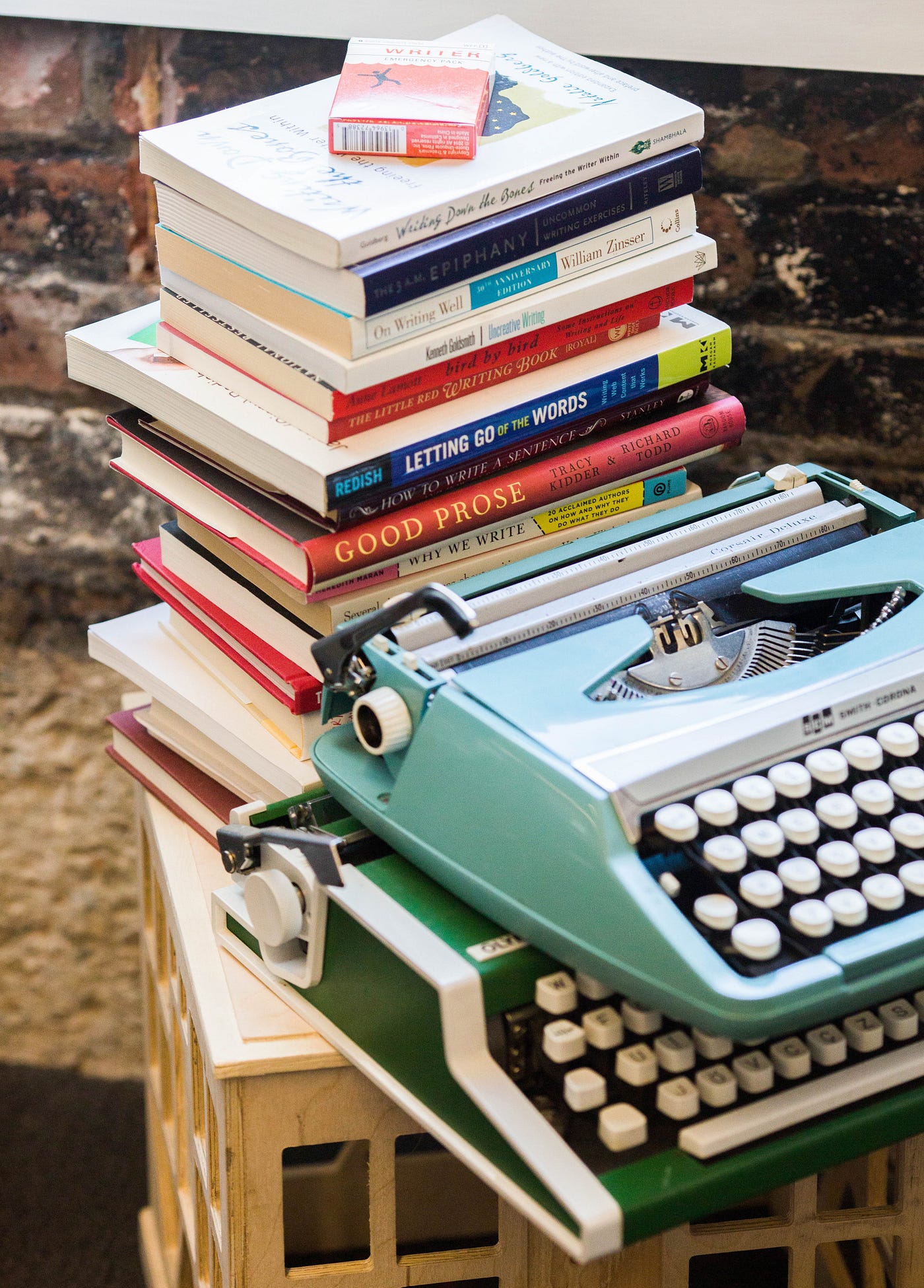This image features a pair of vintage typewriters, one stacked on top of the other, under a wooden structure. The bottom typewriter has a distinct green body with a white border and white keycaps that feature dark black and gray letters. The typewriter on top is a light blue cyan color, also with white keys, though its letters are less discernible and out of focus. Behind the typewriters, there is a tall stack of multicolored books, ranging from shades of white and blue to red. Some of the titles are visible, including "Writer," "Good Prose," "Why We Write," "Letting Go of the Words," and "On Writing Well." These books, taller than the typewriters, are set against an exposed brick wall with a mix of gray, red, and black bricks, suggesting a raw, loft-like setting. The overall scene appears to be a cozy writing nook, with elements like a possible box of chalk or whiteout placed on top of the books. The photograph captures a nostalgic and creative ambiance, reminiscent of a bygone era.